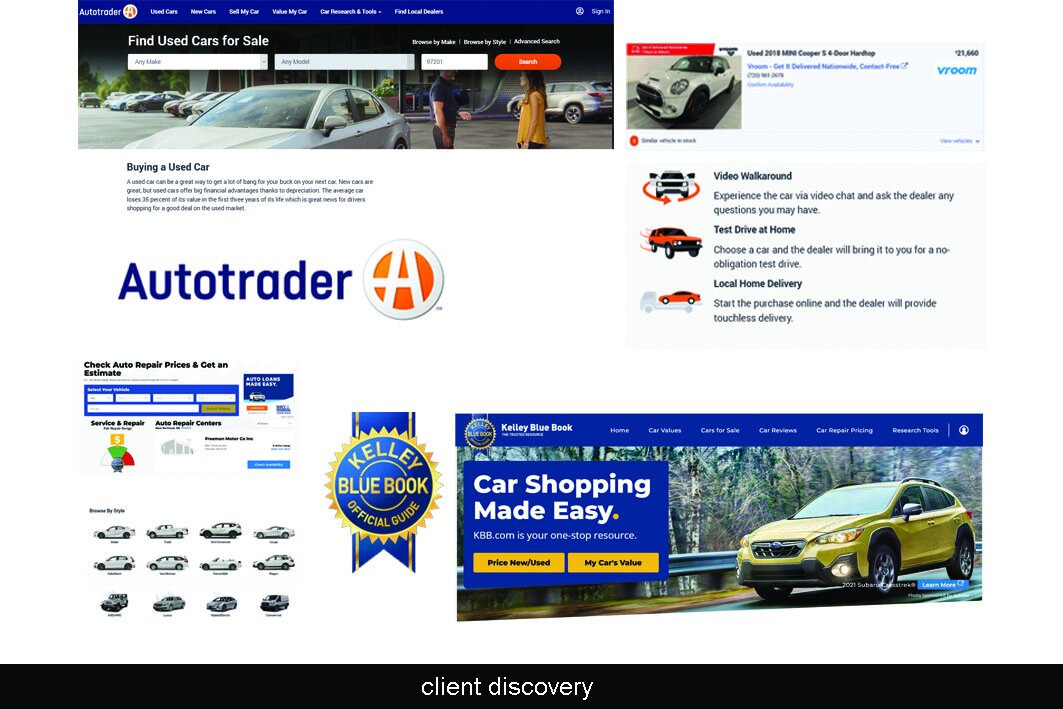This image is a composite screenshot featuring several webpages from the Autotrader brand, arranged in a square format. On the left side, there's a webpage highlighting the option to explore used cars for sale, along with detailed information about the process of purchasing a pre-owned vehicle. On the right side, another webpage displays a used white Mini Cooper with black wheels. This section emphasizes various Autotrader services, including a video walk-around, at-home test drive, and local home delivery options. Notably, it features the official Kelley Blue Book seal, indicating that the company's vehicle valuations are based on Kelley Blue Book data. Additional webpages showcase other services and offerings from Autotrader, rounding out the comprehensive overview of the brand’s features.